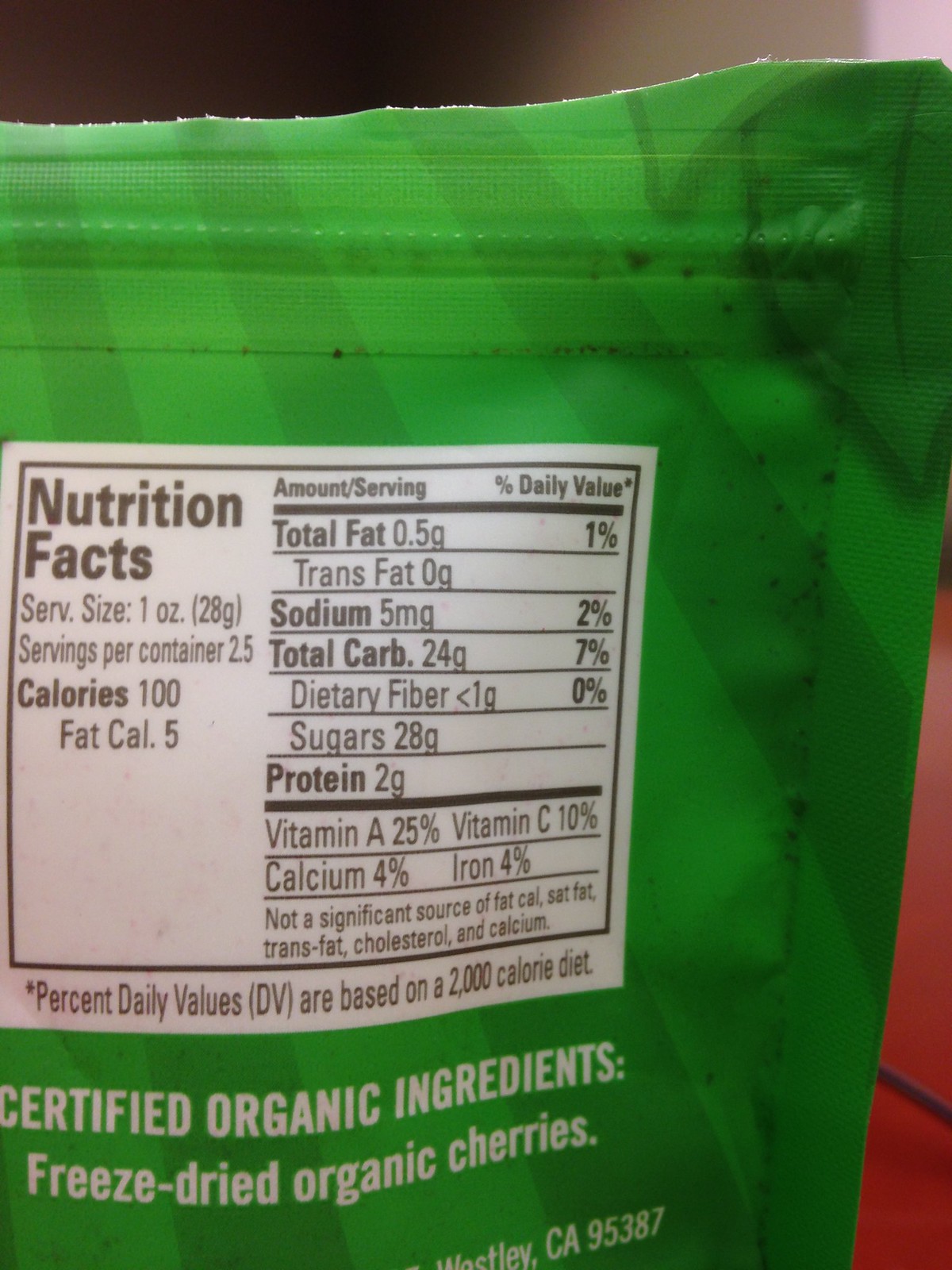This indoor digital photo is a close-up of the back of a bright green bag of freeze-dried organic cherries. The bag features a white square label with detailed nutrition facts in black lettering. The label specifies a serving size of 1 ounce (28 grams) and two and a half servings per container. The nutrition information includes: 100 calories, 5 from fat, total fat 4.5 grams (1% DV), 0 grams trans fat, 5 milligrams sodium (2% DV), 24 grams total carbohydrates (7% DV), less than 1 gram of dietary fiber (0% DV), 28 grams sugar, and 2 grams protein. The label also lists vitamin A at 25% DV, vitamin C at 10% DV, calcium at 4% DV, and iron at 4% DV. Below the nutrition facts, the label highlights in red text that the contents are certified organic ingredients, specifically freeze-dried organic cherries. Additional details, such as the manufacturing location—Wesley, California 95387—are partially visible on the label.